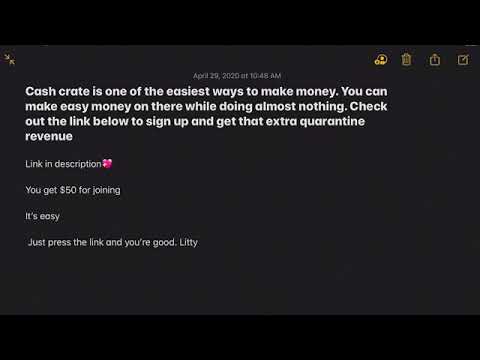The image is a screenshot from a mobile device's note application, centered with no other objects present. The background has a black color with darker black stripes at the top and bottom. At the top right, there are icons for delete, share, and compose, along with a trash can symbol. The date and time, "April 29, 2020 at 10:48 AM," are displayed in a grayish tiny font. The main text in white font reads: "Cash crate is one of the easiest ways to make money. You can make easy money on there while doing almost nothing. Check out the link below to sign up and get that extra quarantine revenue. Link in description ❤️. You get $50 for joining. It's easy. Just press the link and you're good. Liddy." The text is perfectly centered, and there is a small heart symbol next to "link in description." The colors in the image include shades of black, white, dark gray, and a hint of pink from the heart symbol.